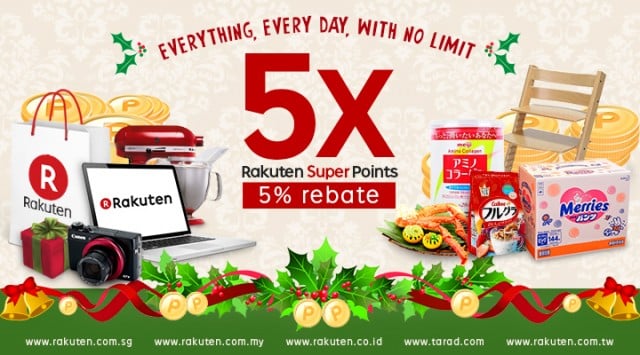The image prominently features a bold red message in all capital letters reading "EVERYTHING, EVERY DAY, WITH NO LIMIT," flanked on each side by two green holly leaves adorned with small red berries in the center. The central eye-catching text announces "5X Rakuten Super Points," with "Super" in red text, followed by "5% Rebate" underneath. To the left side of this central message, there is a vivid image illustrating a red KitchenAid mixer, a bag displaying the Rakuten logo, a stack of gold coins, a laptop branded with Rakuten on its screen, and a Canon camera. On the right side, the imagery includes a box of food, a plate with crab legs, additional gold coins in the background, and a cushioned chair. The bottom part of the image is decorated with more holly intertwined with red ribbon, gold coins embossed with the letter "P," and gold bells at both ends. Below these decorations, various Rakuten website addresses are listed: www.rakuten.com.sg, rakuten.com.my, rakuten.co.id, and rakuten.com.tw.